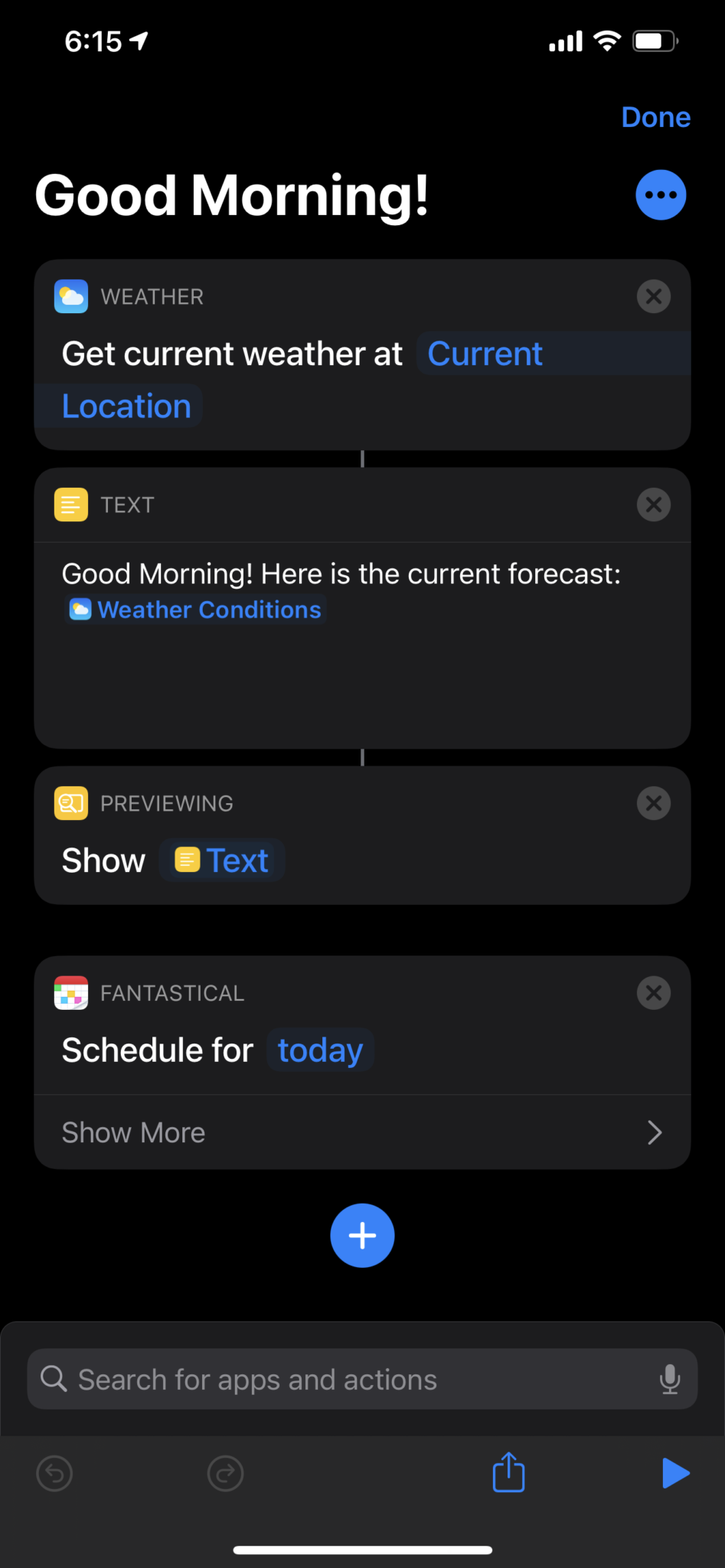The image is a vertical screenshot of a smartphone displaying an app in dark mode. The background is predominantly black. At the top left corner, the time "6:15" is shown, while the icons for battery, Wi-Fi, etc., are displayed on the right. Below these icons in large white font, the text "Good morning" is prominently featured, with a blue "Done" button above it and a blue button with three dots on the right side.

Under the greeting, there's a box for the weather that reads, "Get current weather at current location," with "current location" highlighted in blue, indicating it is a clickable button. Below this, another box labeled "Text" presents the current forecast and includes a blue clickable link for "weather conditions." 

The interface continues in a similar structured manner, with separate boxes for "Preview" and "Fantastical," presumably the user's calendar for the day. At the bottom, a centered button with a plus sign allows for adding new items, and directly below it is a search box flanked by send and upload buttons. The image overall portrays an organized, user-friendly app interface designed for daily planning and weather updates.